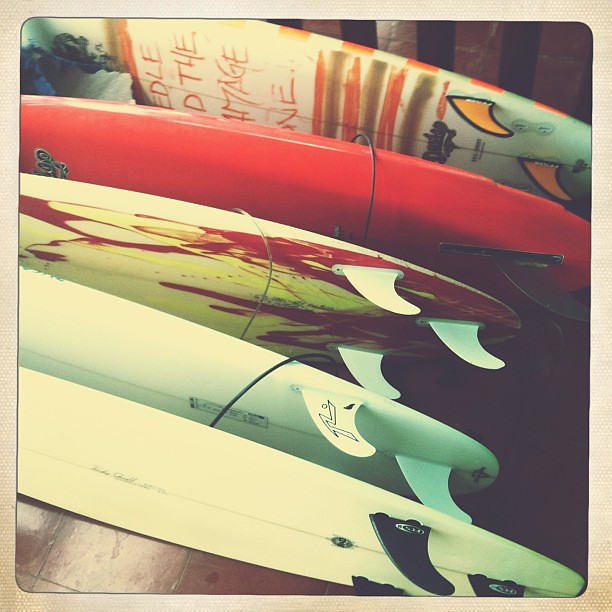The photograph captures an overhead view of five colorful surfboards laying on their sides on a shiny, brown brick pavement. The surfboards are positioned in a row with the ends visible, revealing their three black fins—one on each side and one in the middle. The first surfboard features an abstract orange and brown design with partial orange writing, obscured by the next board. The second surfboard is a striking solid reddish-orange, complete with a black cord wrapped around it. The third board is white with vivid red and yellow ink designs. The fourth surfboard is entirely white and also features a cord. The fifth and final surfboard is solid white but distinguished by its black fins. A stone or masonry wall with slots rises in the background, allowing a sliver of light to illuminate the scene lightly. Framing the image is a brown border that complements the earthy tones of the pavement below.